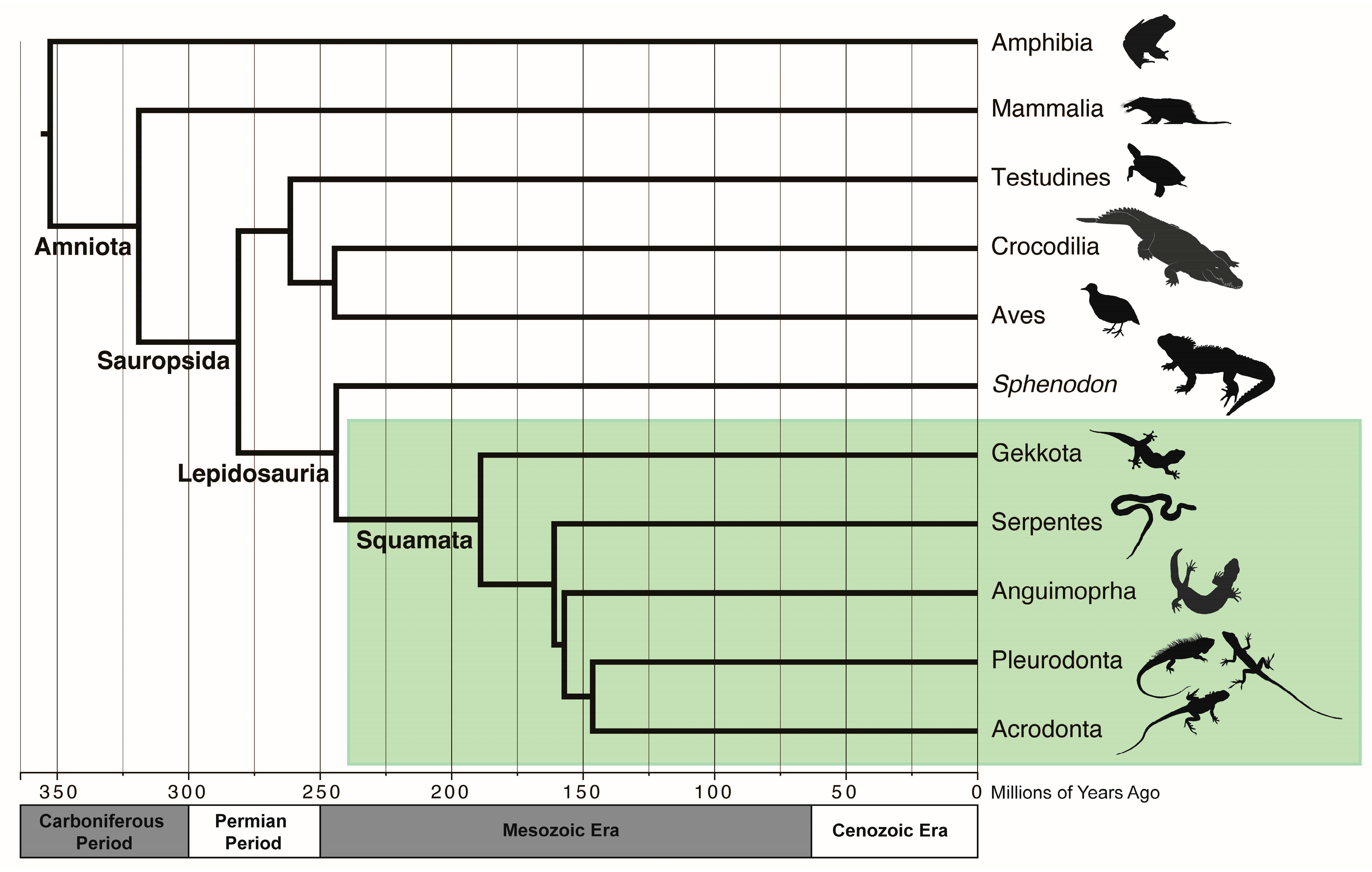The image depicts a detailed evolutionary chart with a white background, showcasing various animal species and their evolutionary timelines. Along the y-axis, there are names and black silhouettes of animals including Amphibia, Mammalia, Testudines, Crocodilia, Aves, Sphenodon, Geckoa, Serpentines, Anguimorpha, Pleurodonta, and Acrodonta. The x-axis measures time in millions of years, ranging from 0 to 350, with different geological periods labeled underneath such as the Carboniferous Period, Permian Period, Mesozoic Era, and Cenozoic Era. Each species has a bar extending horizontally, indicating the period during which it emerged. Notably, there's a section with greenery spanning from Geckoa to Acrodonta, adding a dash of color to the black, gray, and white diagram. No people are present in the image, emphasizing its focus on the evolutionary data.